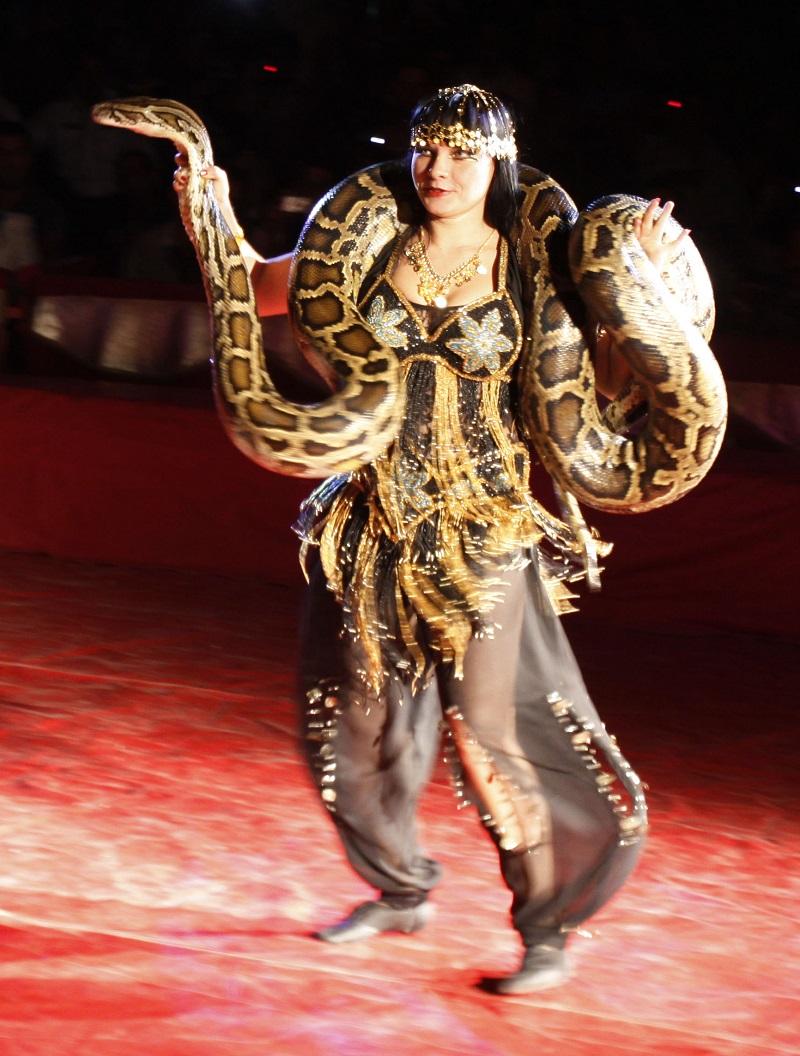This vibrant color photograph captures a young woman dressed as a circus performer, standing on a red floor. She is holding a live, giant python or boa constrictor draped around her shoulders. The snake, as thick as her head, is held firmly in her right hand near its neck and in her left hand by its tail. The woman is adorned in a stunning sequined costume featuring a gold and black top with flower shapes over the breasts, white and green sequins, and a fringed bottom. She complements her ensemble with sheer black pants and black shoes. Adding to her extravagant look is a beaded, sparkling black and gold headdress and an elaborate, jewel-encrusted necklace. The motion blur on the fringe of her top and her feet suggests she is in mid-performance on the circus's red floor, with no other people or structures in the visible background. She smiles as the snake's head remains alert, both facing to the left.